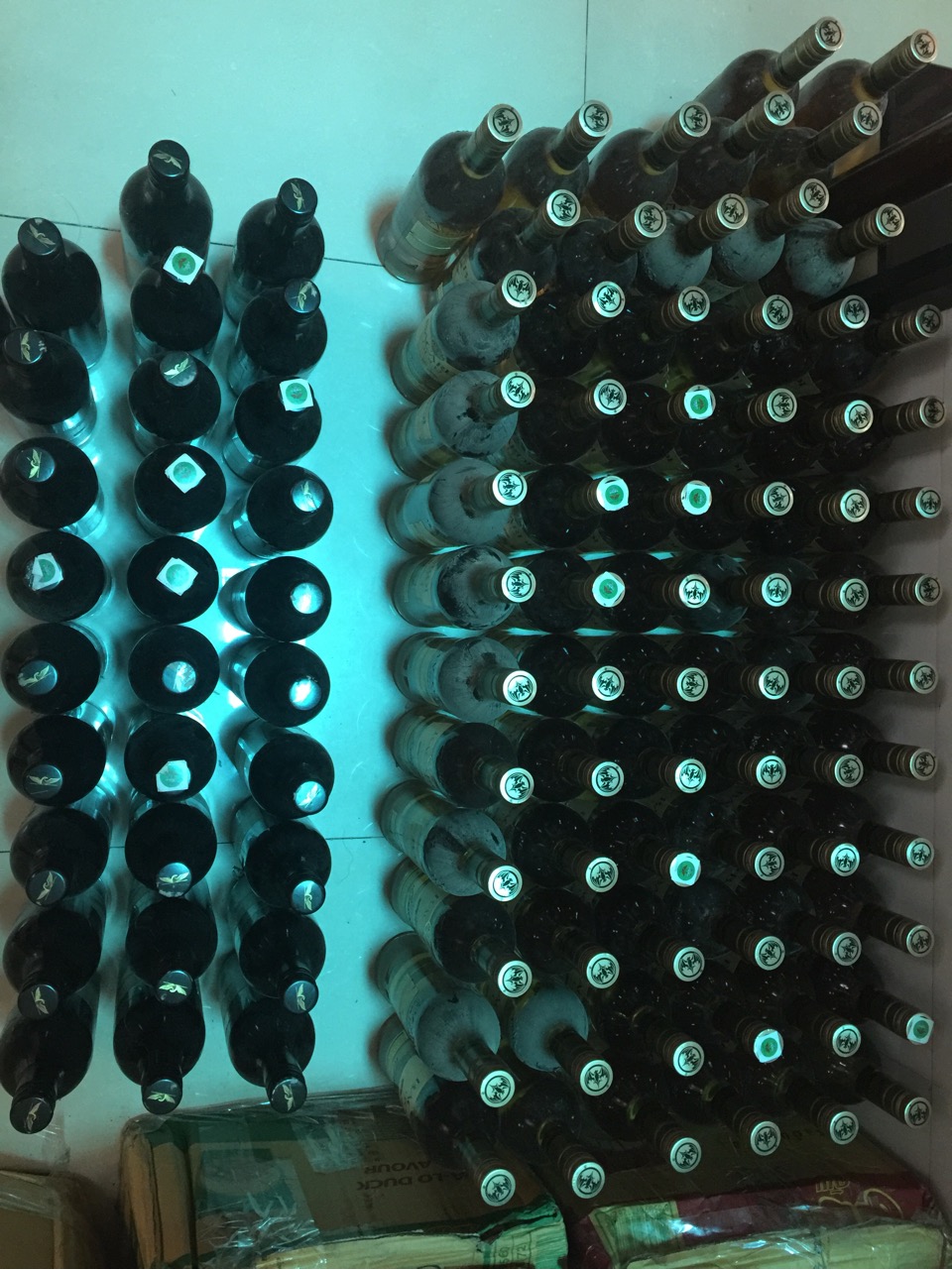This aerial color photograph, with a distinct cyan or blue tint, showcases an organized array of bottles, possibly wine, arrayed on a blue-tinged white tiled floor. The bottles appear to be predominantly standing on their bases with some displaying a noticeable collection of dust, suggesting they were recently retrieved from a wine cellar or similar storage. The caps, highlighted by an overhead light source, feature text and emblems, adding to the uniformity despite varying designs. The overall hue of the image blends blue, black, and bluish-white tones with hints of greenish-brown from the boxes prominently placed at the bottom of the frame, heavily taped and slightly obscured. The right side of the image is densely packed with bottles, which exhibit a mixture of screw-off and possibly corked tops, in contrast to the sparser left side. The neat arrangement and partial visibility of labels enhance the symmetrical pattern, although not all rows are completely filled.